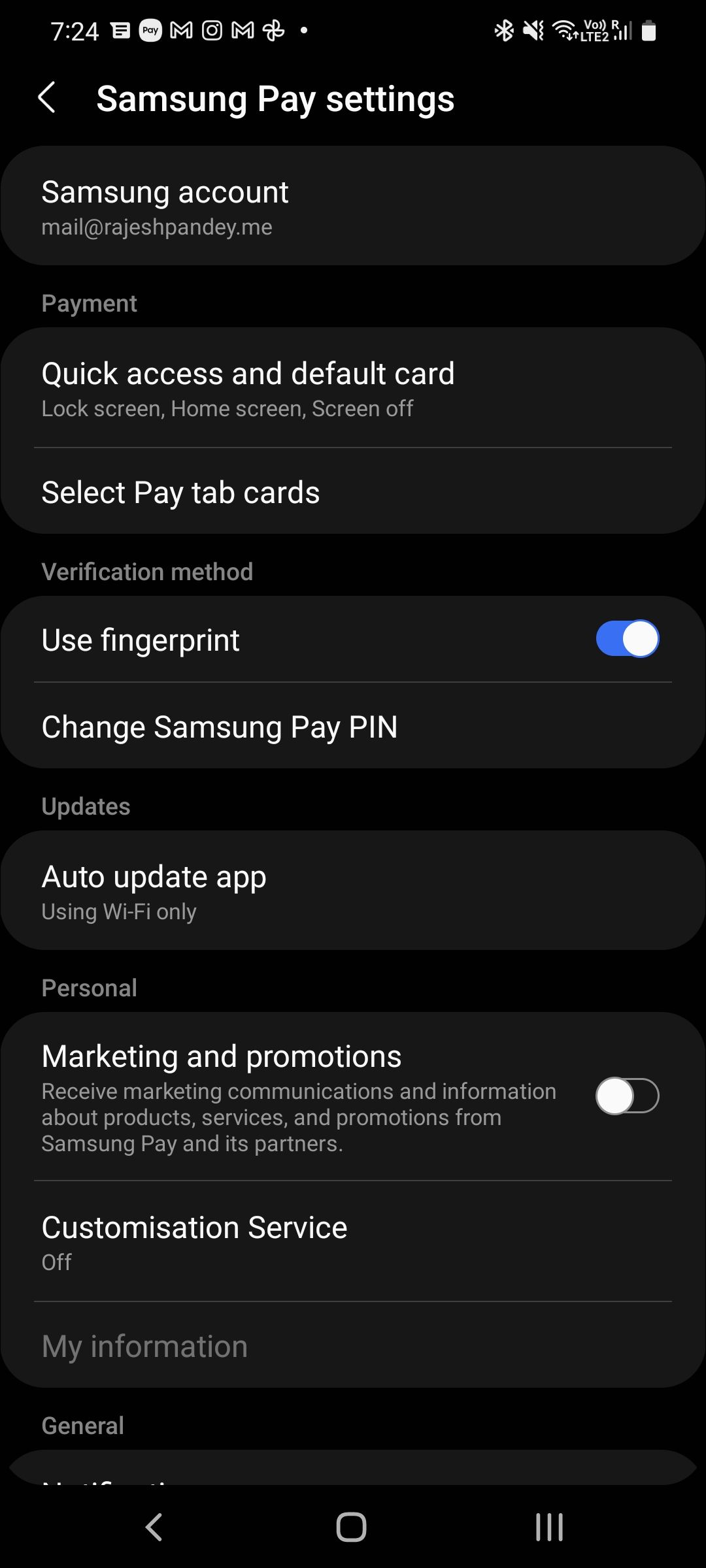The image shows a screenshot of a Samsung Pay settings page on a smartphone. The device's status bar indicates the time as 7:24. A variety of app icons are visible along the top of the screen. The settings page is affiliated with a Samsung account registered to the email "mail@rajeshpandy.me."

Several sections and options are listed within the settings:

1. **Payment**:
    - Quick Access & Default Card
    - Options for accessing Samsung Pay via the lock screen, home screen, or when the screen is off.
    - Selection of payment tab cards.
    - Verification method set to use fingerprint.
    - Option to change Samsung Pay PIN.
    
2. **Updates**:
    - Auto-update app set to "Wi-Fi only".
    
3. **Personal**:
    - Marketing and Promotions: Toggle for receiving marketing communications and information about products, services, and promotions from Samsung Pay and its partners is turned off.
    - Customization Service: The service is turned off, noted by the UK spelling of "customization" with an 's.'

4. **My Information**:
    - This section appears unhighlighted or inactive.

5. **General**.

At the bottom of the screen, there are three navigation icons: a triangle, a square, and a set of three horizontal lines.